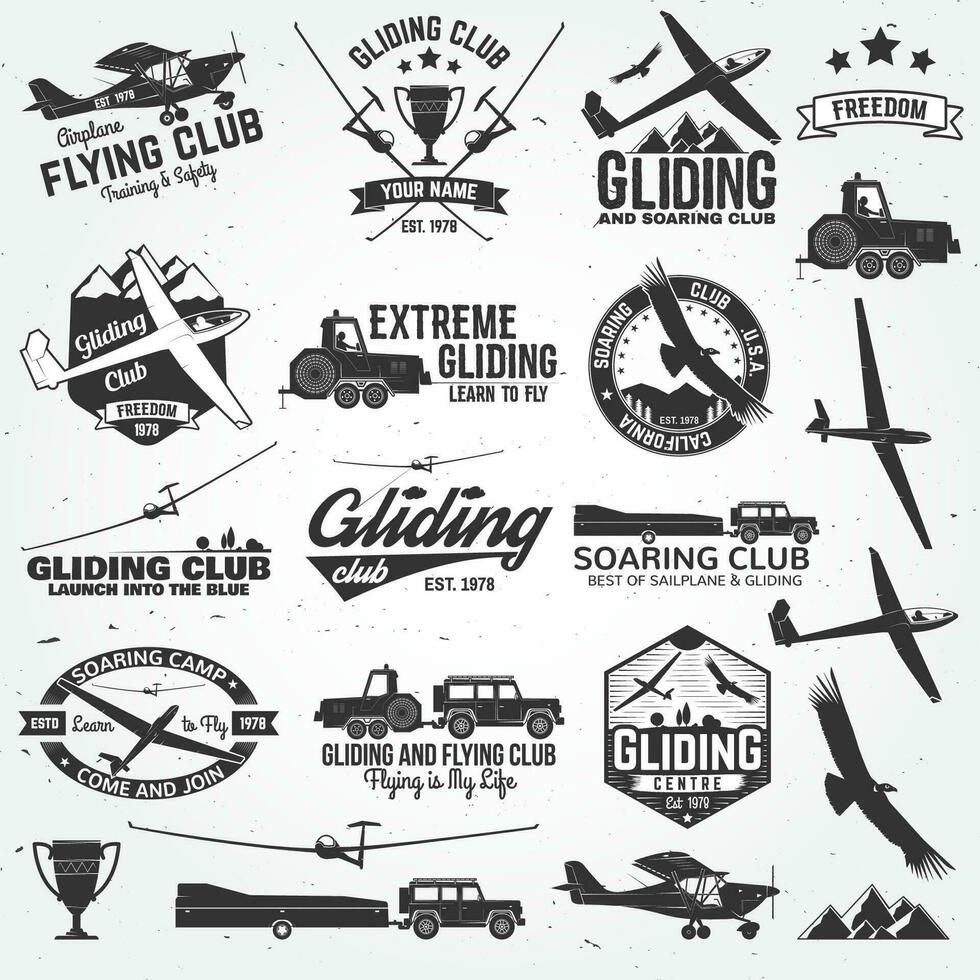The image is a detailed, multi-layered poster on light blue paper, lighter in the center with darker blue around the edges. It features an array of black-and-white logos, mostly centered around different aspects of flying. These include numerous logos from clubs such as the Airplane Flying Club, Gliding Club, Training and Safety, and Gliding and Soaring Club, all established in 1978. Prominent among these are banners that proclaim "Freedom" alongside three stars, logos depicting gliders soaring over mountains, and club names encouraging membership and learning to fly.

The upper left section showcases a plane with black writing underneath, mentioning the flying club. To the right, a trophy with the text "Gliding Club" sits above a customizable name banner with smaller writing below it. Further right is another plane logo labeled "gliding" and then "boring club." Another banner reads "Freedom," accompanied by stars, and beneath it, a tractor or machinery can be seen. 

The poster continues in rows below, with various images including multiple planes, an eagle, and vehicles like a SUV or jeep towing equipment. Each line features combinations of these elements, with a central theme focusing on aviation and gliding achievements, reinforced by logos like "Extreme Gliding Learn to Fly" and "Soaring Club USA California established 1978." Along the bottom, a trophy, a glider, a jeep towing equipment, an old-style plane, and mountain tops are visible, creating a rich tapestry of the gliding community's identity and history.